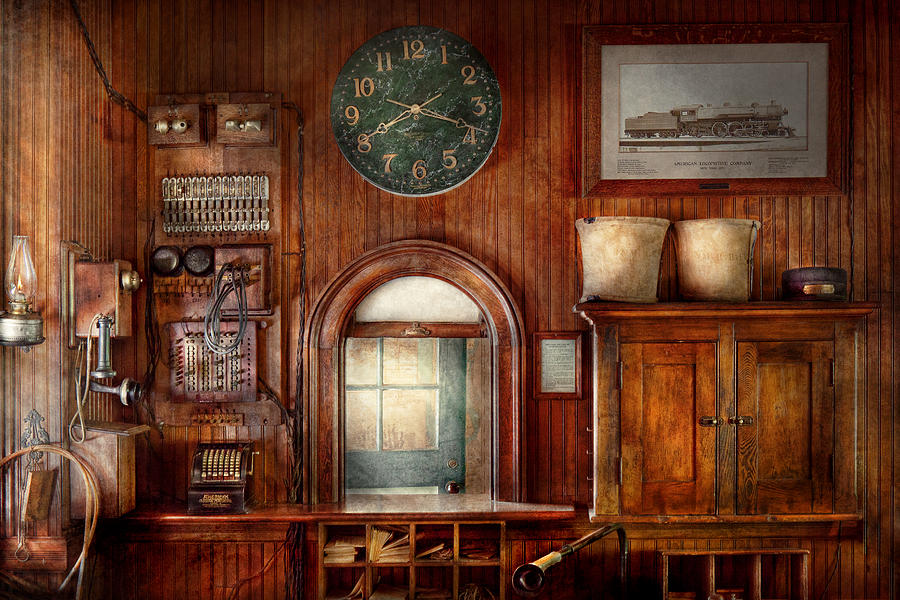This image depicts a wood-paneled room that appears to be an old-time train station or possibly an old general store. Dominating the scene is a large wooden desk with an arched opening that houses a pull-down screen. Beneath this opening, a series of small cubby shelves hold various papers, likely documents or books. Above this setup, an analog clock with gold numbers reading 8:18 is prominently placed, contributing to the room's vintage atmosphere.

To the right of the desk is a wooden cabinet topped with two canvas sacks and a brown sack, alongside a framed text document. A framed image of a train, possibly highlighting the room's connection to railway history, is also located in this area.

On the left side of the room, an array of old-fashioned telecommunication devices can be seen, such as an old-school box telephone with a hanging headset, various switchboards with wires that look like an old-style telephone system, and what might be an old cash register. Adjacent to these, an oil lamp and a rope or lasso hang on the wall. Additionally, items that appear to be a gear mechanism, potentially from a train or an old cash register, add to the historical feel.

Through the window, one can glimpse a door with glass panes directly across, hinting at an exterior or another part of the establishment. The room, rich in wooden surfaces and historical artifacts, evokes a strong sense of a bygone era, possibly when train travel was a dominant mode of transportation.